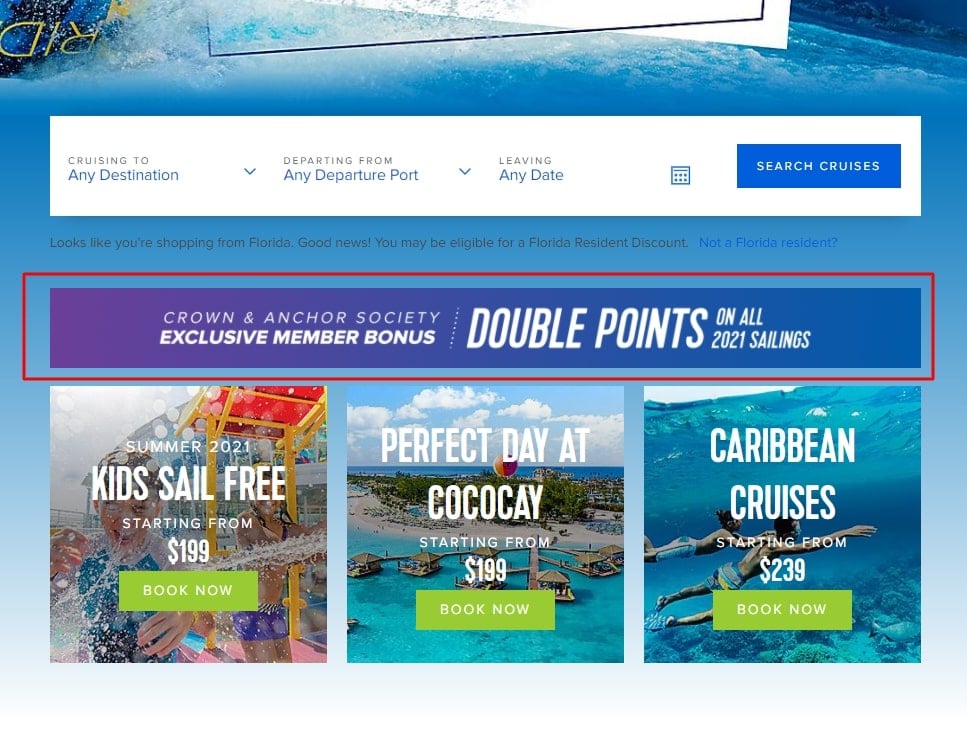Screenshot of a travel website highlighting a promotional banner offering "Crown and Anchor Society Exclusive Member Bonus: Double Points on All 2021 Sailings." The banner features a gradient that shifts from purple on the left to blue on the right. The mobile page has been scrolled down, obscuring the main website title. The background of the UI depicts a pool's interior view, looking upward towards the crashing waves above.

The website showcases options to search for cruises based on three criteria: destination, departure port, and departure date. Additional promotions highlighted include special offers for Florida residents, summer 2021 kids sailing free starting from $199, a "Perfect Day at CocoCay" package starting from $199, and Caribbean cruises starting from $239, with "Book Now" buttons accompanying each offer.